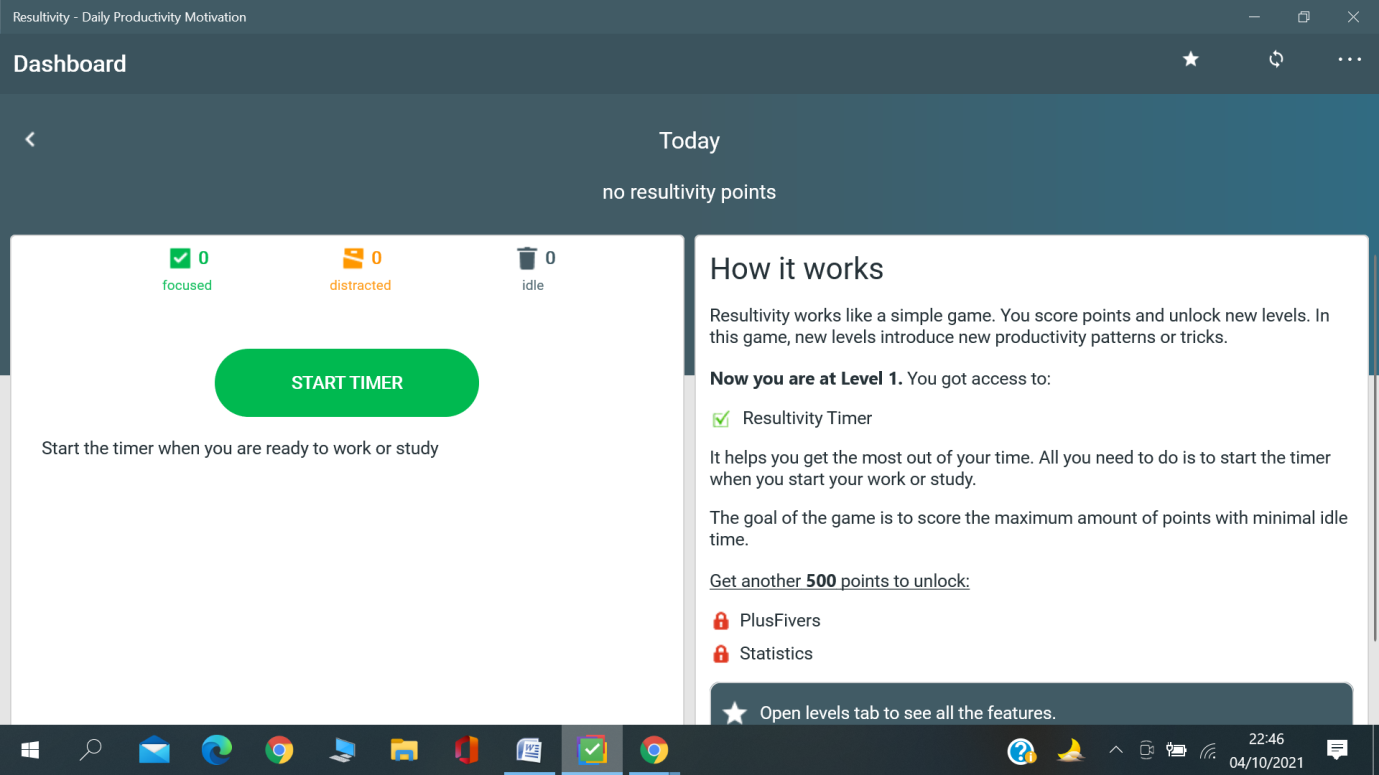The webpage features a medium blue background with a slightly darker blue at the top. On the left side of the top bar, it reads "Resultivity / Daily Productivity Motivation." On the right side, there are three icons: a hyphen, a square, and an "X." 

Just below this is a darker blue banner that says "Dashboard" on the left. On the right side of this banner are three symbols: a star, a circle of arrows, and three dots.

In the middle of the medium blue background, there is a heading that says "Today" followed by "No Resultivity points." Below this, on the left, is a large white square. Inside this square, there are three sections indicating different statuses: 
1. A green square with a white checkmark labeled "Focused" with a zero next to it.
2. An orange square with a white line labeled "Distracted" with a zero next to it.
3. A gray trash can labeled "Idle" with a zero next to it.

In the center of this white square, there is a button labeled "Start Timer" and a note below it saying, "Start the Timer When You Are Ready to Work or Study."

To the right of this is another large white square labeled "How It Works." This section explains that Resultivity operates like a simple game where points are scored, and new levels are unlocked, introducing new productivity patterns or tricks. It mentions that currently, the user is at level 1 and has access to the Resultivity Timer, which helps maximize productive time. The goal is to score the maximum points with minimal idle time, and it encourages getting another 500 points to unlock Plus Fibers Statistics.

Below this is a partially visible blue square with a white star that says, "Open Levels tab to see all the features."

At the bottom of the webpage is a black banner containing various icons: a window, a magnifying glass, an envelope, a blue swirl, the Google icon, a laptop (possibly), a file folder, an orange square, a white square, a green square with a white checkmark in it, the Google icon again, a blue square with a white question mark, a crescent moon, an upward arrow, a video camera, an unknown icon next to the video camera, a signal strength icon, the number sequence 224604102021, and a white chat box next to it.